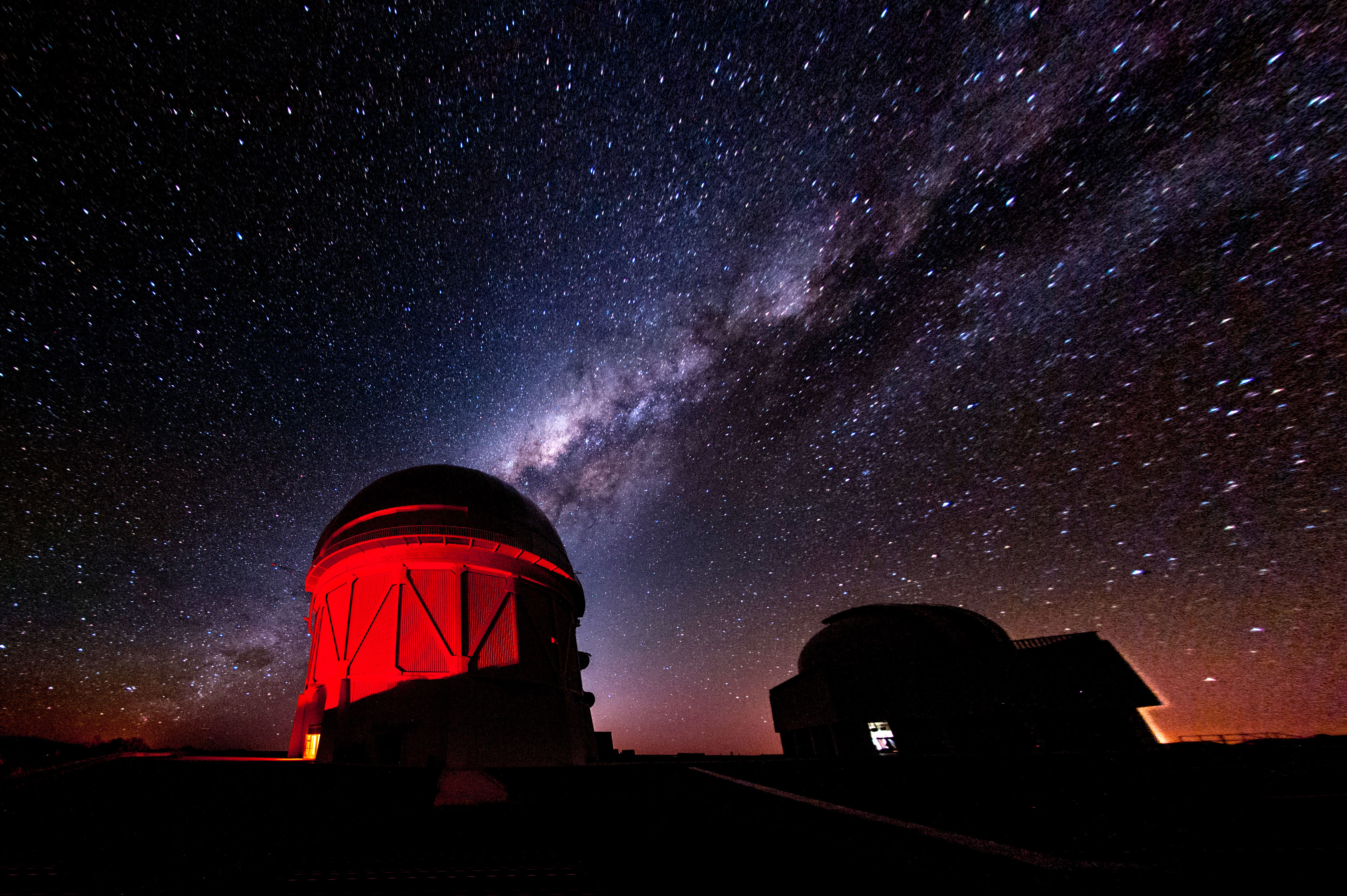The image features a breathtaking nighttime landscape with a sky filled with an innumerable amount of stars, reminiscent of scenes from a movie. The horizon at the bottom of the photo is shrouded in darkness, with a subtle glow suggesting the sun either has just set or is about to rise. In this tranquil setting are two buildings: on the right, a relatively featureless, rectangular structure with a dome, shrouded in darkness and barely distinguishable. On the left, a taller cylindrical building with a dome illuminated by a striking red light. This illuminated structure appears to be an observatory, likely housing a telescope. The two buildings stand out starkly against the brilliantly star-lit sky, which is devoid of any city light pollution, allowing deep colors and light purples to be visible among the stars. The scene exudes a calm and serene atmosphere, emphasizing the beauty and stillness of the night.